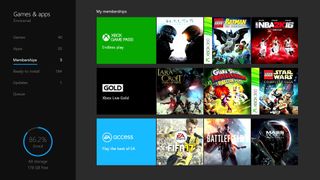This image is a blurry screenshot from an Xbox interface. On the left side, there is a vertical banner in dark black labeled "Games and Apps" at the top, followed by several unreadable categories underneath. One of the highlighted sections appears to be labeled "Memberships," indicating the current page. A progress circle on this page displays roughly 96.2%, though its exact meaning is unclear.

Towards the right, occupying around 75-80% of the screen, is a darker gray background with the heading "My Memberships" positioned towards the top left. Below this heading, several game icons are displayed. Some of the visible games include the green Xbox logo, Lego Batman, NBA 2K16, Lego Star Wars, Lara Croft, Battlefield, FIFA, and potentially Halo. The games feature a variety of characters, from Lego figurines and superheroes to soccer and basketball players, creating a diverse visual representation of available memberships and games.